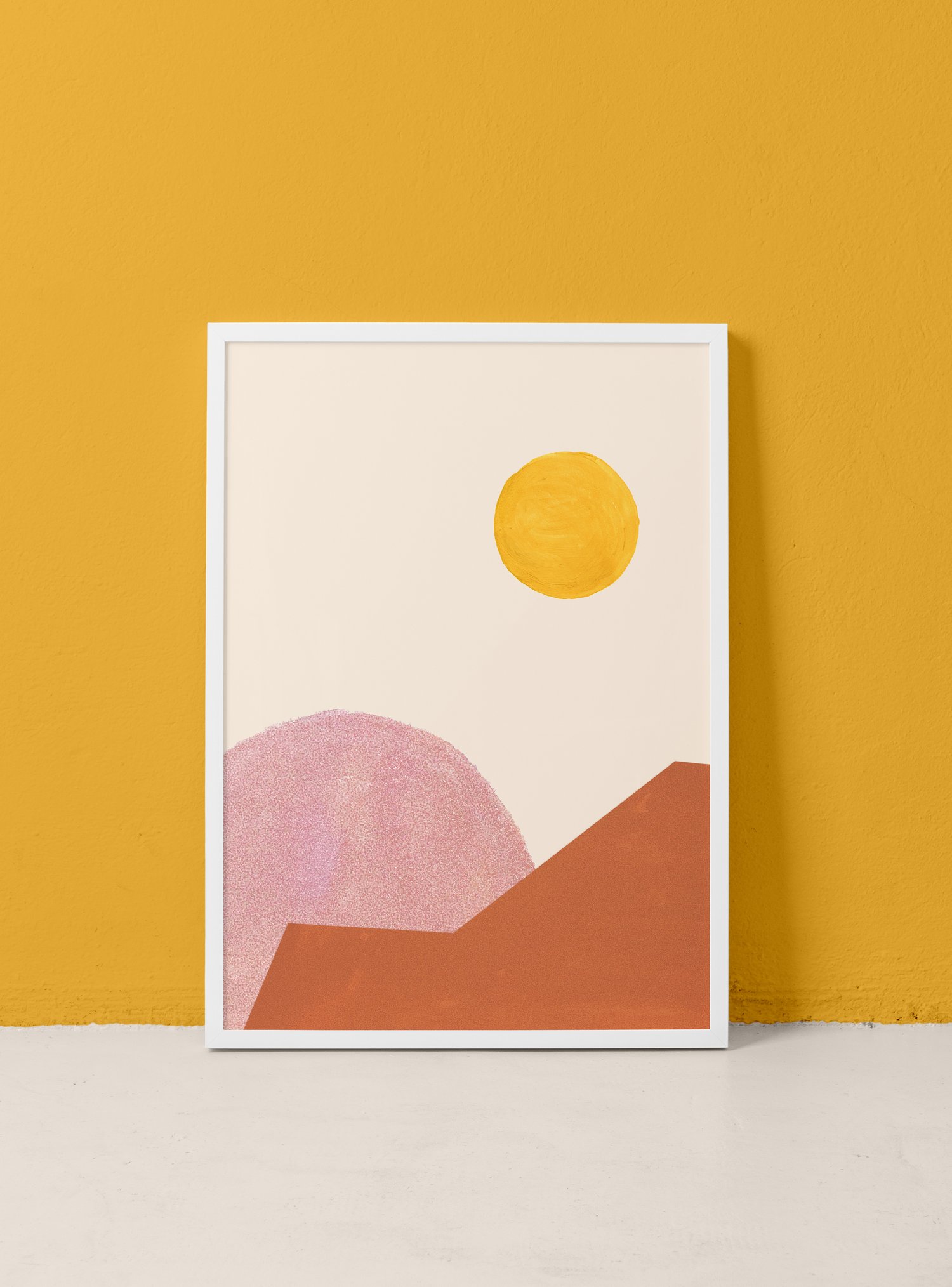The photograph captures a minimalist painting leaning against a vibrant mustard yellow concrete wall, which casts a shadow, implying natural light. The painting itself is encased in a white wooden frame and rests on a stark white concrete floor. The composition of the painting is simple, featuring predominantly three colors: yellow, brown, and pink. The top right corner showcases a yellow circle, symbolizing the sun in an off-white sky. The foreground mountain, painted in a brown hue, and a linear, brick-red structure are found at the painting's bottom, overlapping a pink semi-circle shape occupying the lower left corner. This streamlined art piece exhibits a blend of natural and geometric elements, framed harmoniously within its limited color palette.